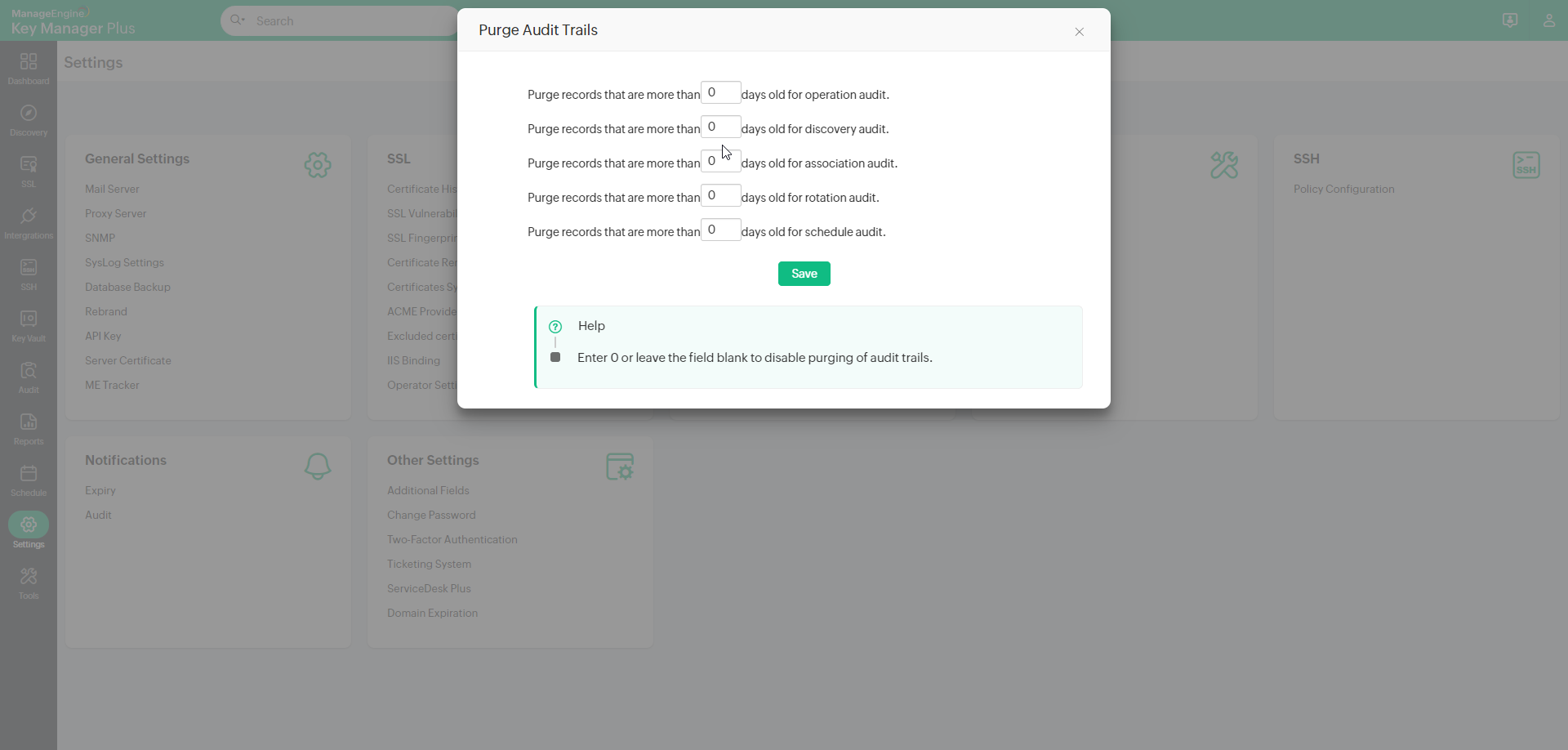The webpage displays a user interface for "Key Manager Plus" by Manage Engine. At the top left of the screen, "Manage Engine" is prominently displayed, with "Key Manager Plus" written in a larger font below it. On the top right side, there is a search bar available.

Below the header, a dark gray vertical menu is located on the left side of the screen. This menu features white icons and text, starting with "Discover" at the top, followed by several other icons that are not clearly readable. At the bottom of this vertical menu, there is a green section labeled "Settings" accompanied by a white icon.

To the right of this vertical menu, there is a comprehensive list of settings and management options. These include: 
- User Management
- General Settings
- Privacy Settings
- Purge Audit Tools
- Export Settings
- Export Data Settings
- Email IDs
- SSH
- SSL
- Notification
- Additional Fields
- Change Password

On the far right side of the screen, a section titled "Purge Audit Trails" is displayed. This section lists five rows under the heading "Purge Records that are more than ____ days old," each accompanied by a box where users can enter a number. The categories listed are:
- Operation Audit
- Discovery Audit
- Association Audit
- Notation Audit
- Schedule Audit

Below these options, there is a green "Save" button. At the bottom, explanatory text reads, "Help: Enter Zero or Leave Field Blank to disable purging of audit trails."